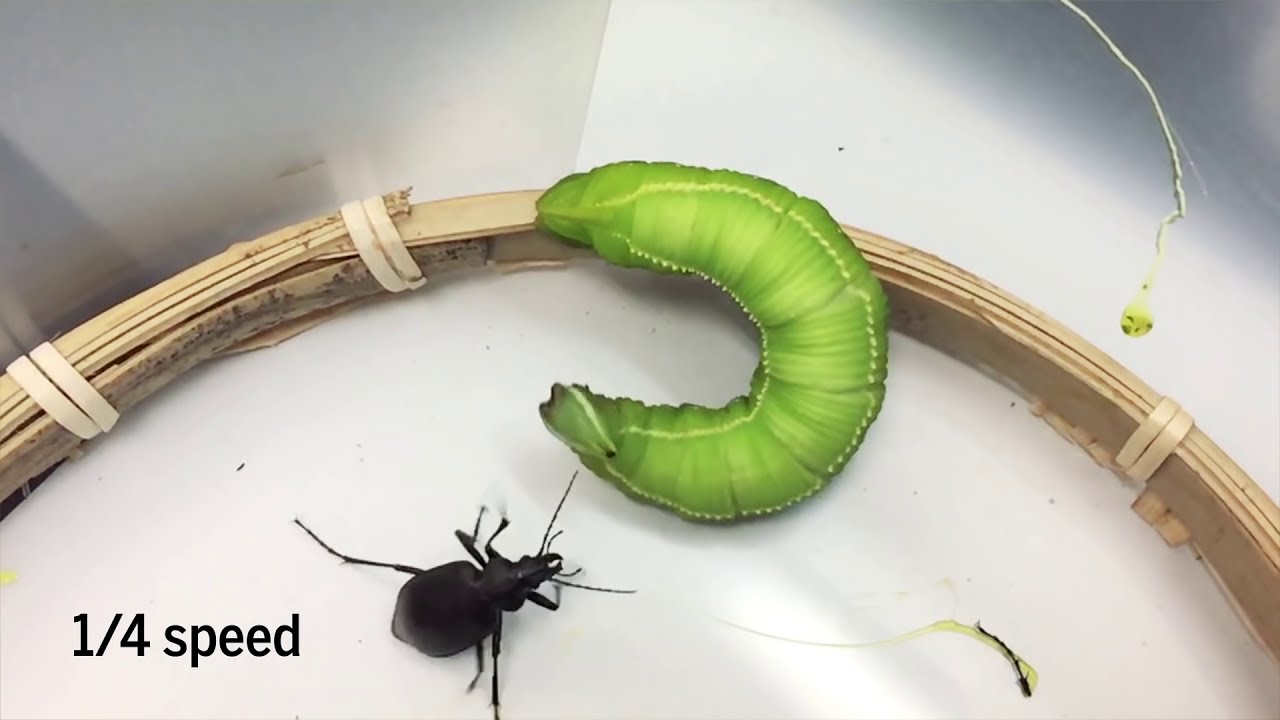In this detailed image, we see a scientific setting where two insects are enclosed in a container. The bottom of the image features a dark-colored bug, possibly a roach, with a large rear end, narrow midsection, and front-facing sharp pinchers, accompanied by six long legs and antennae. Above it, a vibrant green caterpillar-like insect takes center stage, curving into a C-shape towards the left. This creature is characterized by its lime green body adorned with tiny white spiky points along both sides. The environment inside the container includes a platform made of bamboo sticks, bound together with a rubber band, creating a structured base. The background is a shiny silver wall, giving a confined yet distinct setting for both insects. Text in the lower left corner reads "1/4 speed," adding a layer of scientific observation to the scene. Various colors such as white, black, shades of green, yellow, and brown prominently feature throughout the image.